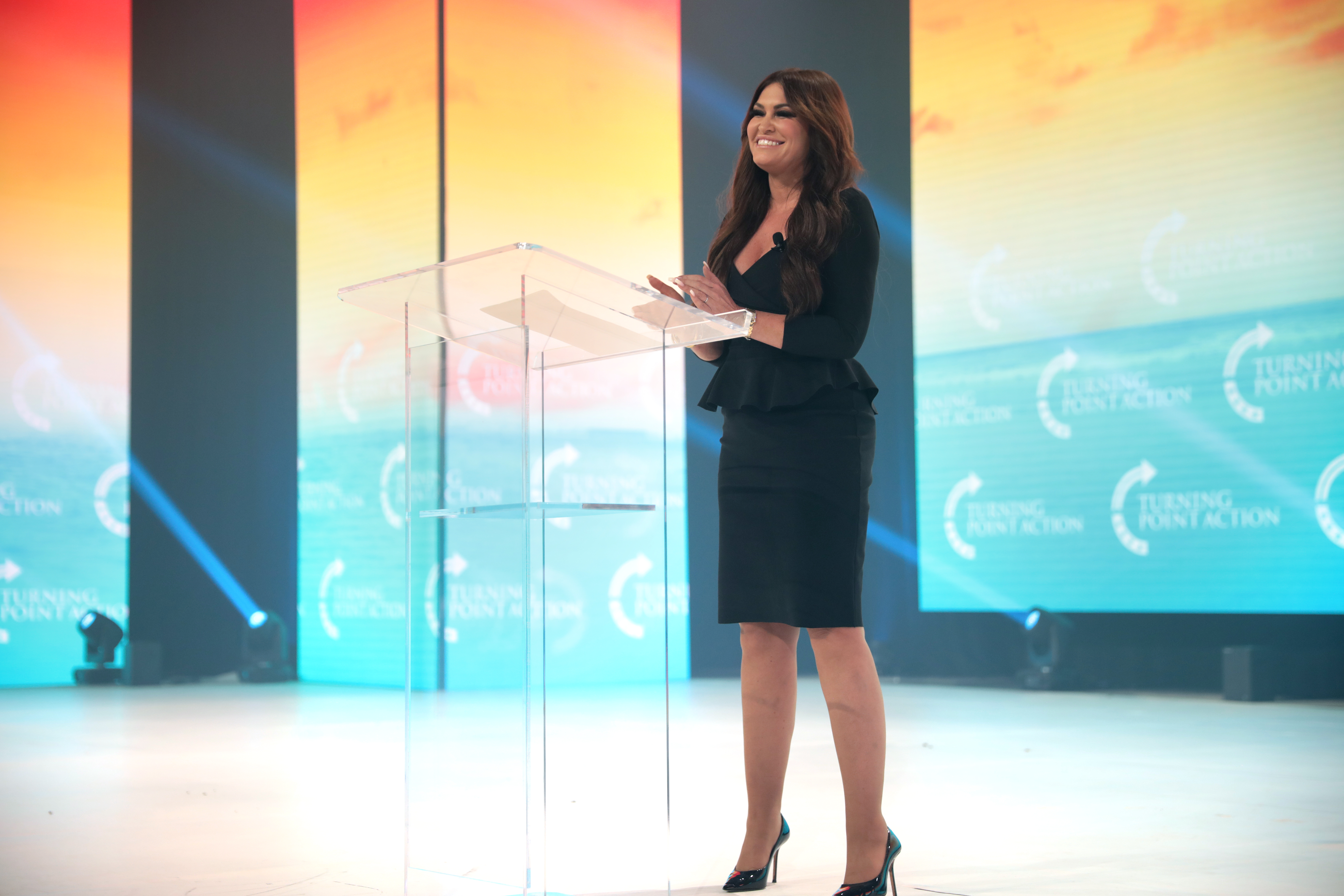The photograph captures a woman standing confidently on a stage, addressing a crowd with a delighted expression. She's attired in a dark blue or black suit paired with black high heels. Her long, dark hair cascades down past her shoulders, and she appears to be smiling, her hands possibly in a clapping motion. The stage is illuminated by several spotlights, and a sleek, all-glass podium stands before her with a piece of paper on it. Behind her, large video screens display an orange and turquoise backdrop with the words "Turning Point Action" and an arrow semicircle logo. Despite a minimalistic setting with no other visible people, buildings, or vehicles, the atmosphere is electrifyingly vibrant, emphasizing her prominent presence at the event.